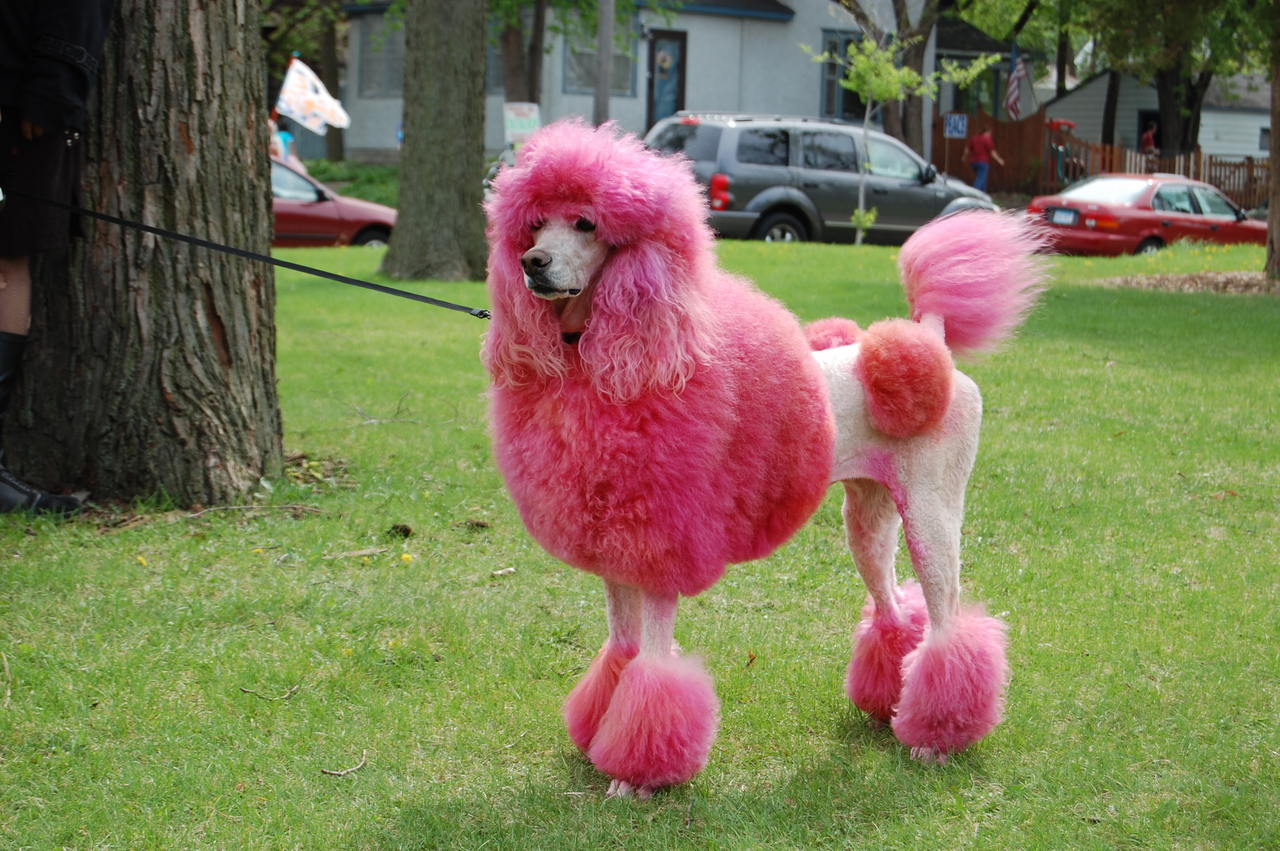This photograph captures a whimsical and somewhat humorous scene set in a lush, green grassy area. At the center of the image stands a poodle, which immediately draws attention due to its unusual and striking appearance. The poodle’s body is mostly white and closely shaved, but it features several distinctive pink elements that give it an extravagant look. The paws are decorated with fluffy pink pom-poms, and the dog's tail is similarly adorned in pink. The upper half of its torso is covered in pink fur, resembling a fur coat, and it appears to be wearing a pink wig – though it’s unclear whether these are part of an elaborate grooming style or attire.

The dog is on a black leash that extends out of the frame, indicating that its owner is just outside the field of view. In the background, there are scattered trees and a line of parked cars, with residential houses visible across the street, suggesting that this photo was taken in a park or a similar open public space. The overall image evokes a sense of humor and curiosity due to the striking contrast between the poodle's natural white fur and the exaggerated pink enhancements, making it appear as though the dog is enveloped in a cloud of cotton candy.